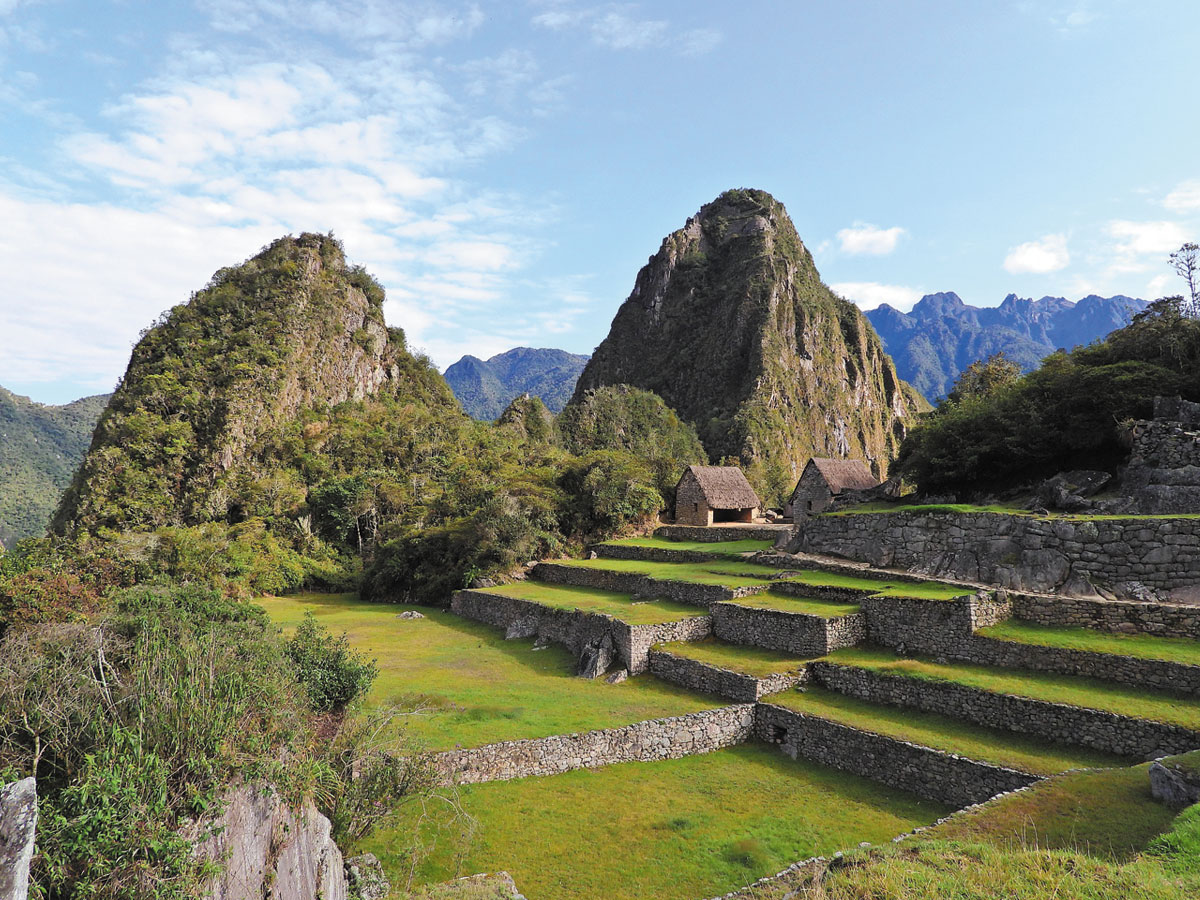The photograph depicts an ancient Incan-like village nestled within a lush, mountainous landscape. Prominent stone terraces, now overgrown with grass, stretch across the scene, creating a stepped appearance that blends harmoniously with nature. In the foreground, the terraced stone structures, although aged, retain a sense of timelessness. Towards the rear, two small, yet well-preserved houses with thatched roofs and peaked stone walls stand prominently, providing a glimpse into the village's architectural ingenuity. Beyond these structures, the landscape extends into rolling hills adorned with abundant foliage, and further in the distance, a range of majestic mountains can be seen under a vibrant blue sky scattered with fluffy white clouds. The image emanates a serene beauty, highlighting the intricate relationship between human craftsmanship and the untamed wilderness.